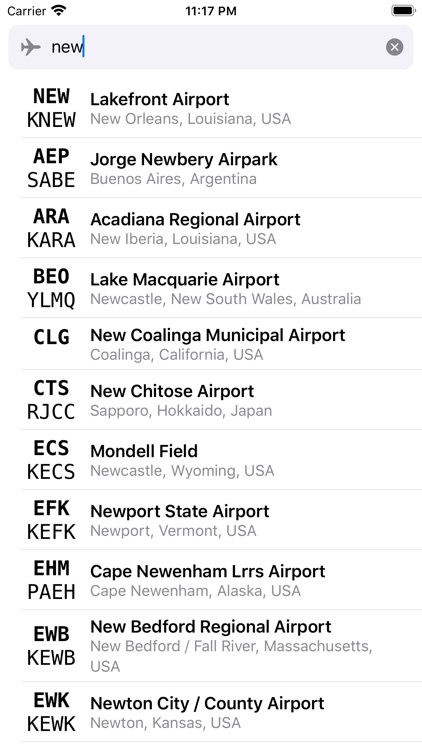Here is a detailed and cleaned-up caption for the provided image:

---

The image is a smartphone screenshot displaying a list of airport codes and names. At the top, the screen shows a status bar with a carrier signal, Wi-Fi icon, the time "11:17 p.m.," and a fully charged battery icon. Below the status bar, an airplane mode icon is visible. 

The main content consists of a search bar where the word "NEW" has been typed in, with a sky blue cursor positioned at the end of the word. To the right of the search bar is a closeout "X" icon. Beneath the search bar is a list of entries in vertical order, detailing various airports containing the term "NEW":

1. "NEWKNEW" - Lakefront Airport, New Orleans, Louisiana, USA.
2. "AEP/SABE" - Jorge Newbery Airport, Buenos Aires, Argentina.
3. "ARA/CARA" - Acadiana Regional Airport, New Iberia, Louisiana, USA.
4. "BOYLMKQ" - Lake Macquarie Airport, Newcastle, New South Wales, Australia.
5. "CLG" - New Coalinga Municipal Airport, Coalinga, California, USA.
6. "CTSRJCC" - New Chitose Airport, Sapporo, Hokkaido, Japan.
7. "ESCKECS" - Mondell Field, Newcastle, Wyoming, USA.
8. "EFKKEFK" - Newport State Airport, Newport, Vermont, USA.
9. "EHMPAEH" - Cape Newenham LRRS Airport, Cape Newenham, Alaska, USA.
10. "EWBKEWB" - New Bedford Regional Airport, New Bedford/Fall River, Massachusetts, USA.
11. "EKWKEWK" - Newton City/County Airport, Newton, Kansas, USA.

Each entry lists an airport code followed by the airport's name and location, organized by city, state, and country.